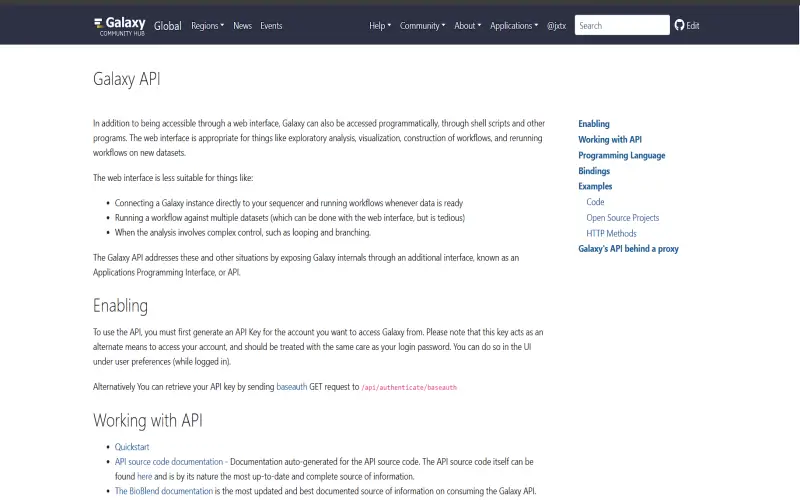**Caption:**

A detailed screenshot showcasing the Galaxy API website. The website's design predominantly features a white background paired with black text on the left-hand side and blue text on the right-hand side. At the top of the page, there is a dark grey navigation bar containing several tabs, including Global, Legions, News, Events, Help, Community, About, and Applications.

On the upper left corner, a search bar is displayed, with a text box and a microphone symbol adjacent to it, labeled "Edit" in white text. Below this, the main heading "Galaxy API" is prominently visible in black text, followed by a subheading titled "Enabling" and another paragraph.

Further down are clickable blue text links such as Quick Start, API Source, Code, Documentation, and Bow Blend Documentation, which offer easy access to various resources. Additionally, a pink link directs users to the "API Authenticate" section. 

On the right side of the image, there are more links, including Enabling, Working with API, Programming Language Bindings, Example Code, Open Source Rights, and HTTP Methods, providing users with a wide array of informational and technical options.